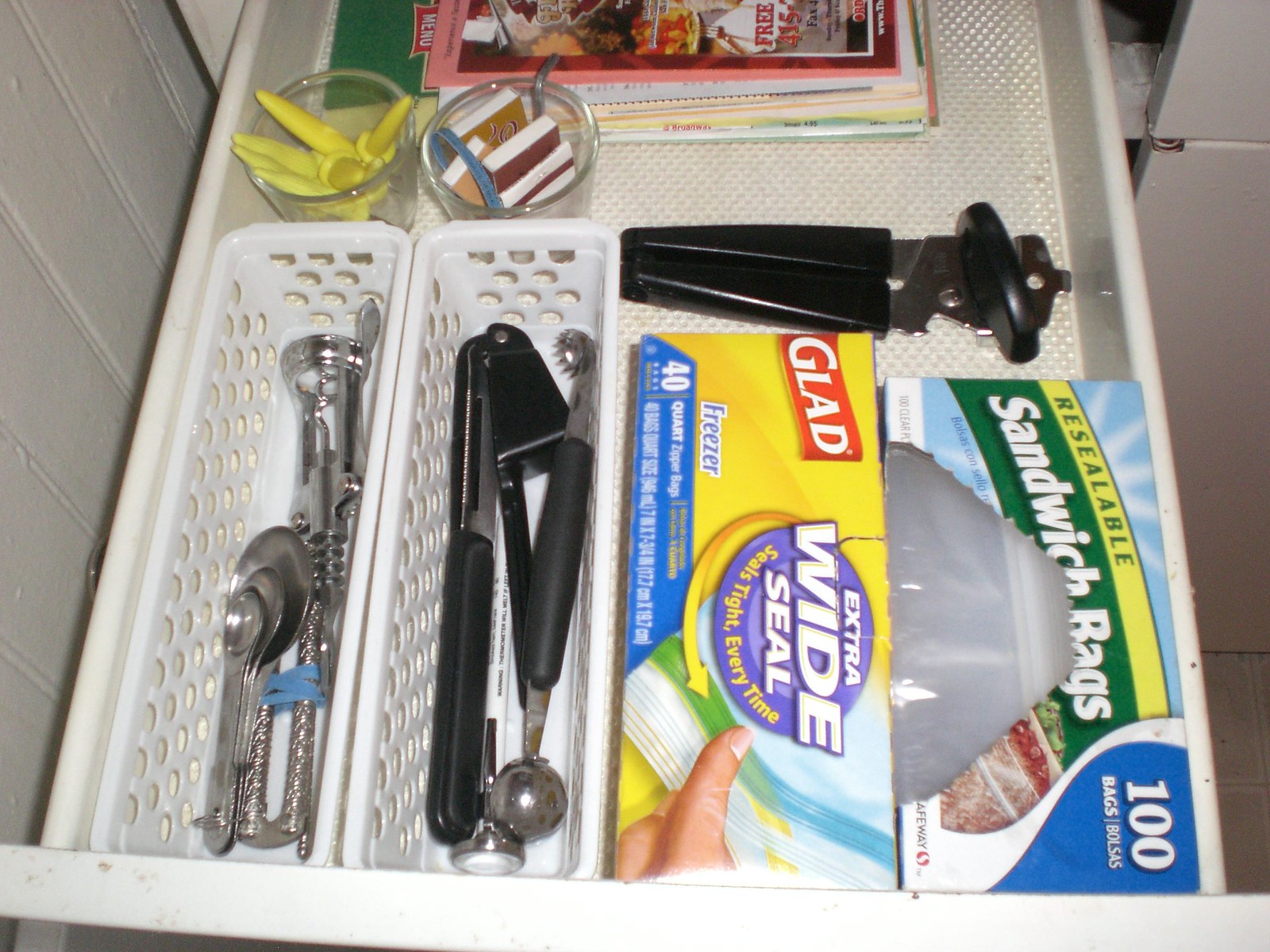The image depicts the meticulously organized interior of a kitchen drawer, which is housed within a white cabinet that seamlessly blends into the white paneled wall. The pristine white drawer is lined with protective paper to prevent scratching. At the back of the drawer, several booklets are neatly arranged; these could include restaurant menus or compact phone books. In front of these booklets, two thick glass shot glasses serve a utilitarian purpose: one is filled with yellow corncob picks, designed for holding corn without getting buttery fingers.

Adjacent to the shot glasses, a small assortment of either notebooks or matchbooks is positioned, with a can opener lying next to them. At the forefront of the drawer, on the right side, there are two boxes of storage bags. The rightmost box contains 100 Safeway sandwich bags, featuring an image of a partially sealed sandwich. Next to it is a box of Glad Extra Wide Seal quart-sized freezer bags, with a depiction of a hand sealing the bag securely.

To the left of the storage bags, two rectangular storage caddies are neatly placed. One caddy contains items such as a meat or food thermometer, a melon baller, and possibly a knife. The identical caddy beside it holds measuring spoons and a corkscrew for wine bottles. This detailed glimpse into someone's organized kitchen drawer exemplifies orderliness and functionality, showcasing a thoughtful arrangement of various kitchen tools and supplies.